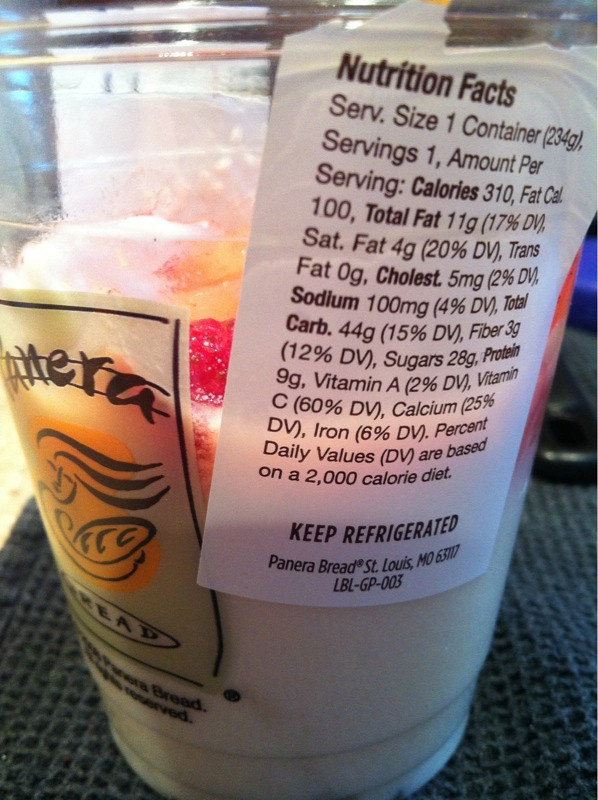A detailed photograph captures a Panera Bread beverage or yogurt placed inside a transparent white cup. The Panera Bread logo is visible on the left side of the cup, which is turned partially away from the viewer. The cup is resting on a gray kitchen dish rag with a distinct waffle texture, reminiscent of a waffle-knit shirt. 

Prominently displayed on the cup is a white nutritional facts sticker with black text, detailing information such as 310 calories, 11 grams of total fat, 5 milligrams of cholesterol, 100 milligrams of sodium, 44 grams of carbohydrates, and 9 grams of protein. However, the sticker does not specify the exact contents of the cup. The text advises to keep the contents refrigerated. 

Half-filled, the cup appears to contain a creamy white substance, likely yogurt, topped with assorted fruit pieces. Visible fruits include a raspberry and an indistinct orange piece, which might be pineapple. The background is somewhat blurred but shows a black object, possibly a remote control, and a blue light likely emanating from a television screen.